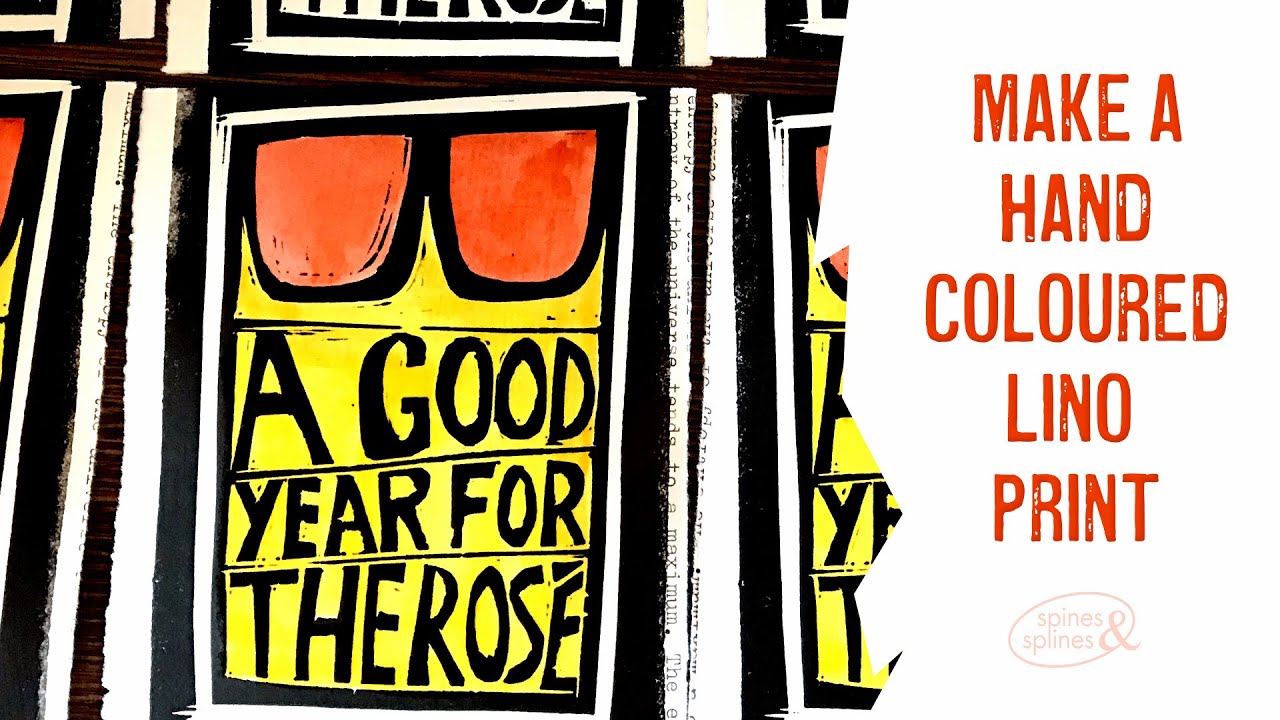The multi-colored print piece is a horizontally rectangular image divided into two distinct sections. The right side is white with jagged edges on the left, resembling torn paper, and features red, capitalized text saying, "MAKE A HAND-COLOURED LINO OR LINO PRINT," highlighting the British spelling of "colored." In the lower right corner of this white section rests an oval logo with an orange border, reading "Spines and Splines."

The left two-thirds of the image showcases an example of a linocut print overlaid on a text background, though the text is mostly obscured by the artwork. The linocut print features large, variable-thickness black lines and several vertical lines of different weights. Centrally positioned within this area is a black-bordered, yellow box containing orange-tinted sunglasses at the top and black text reading, "A GOOD YEAR FOR THE ROADS." This design element repeats in part on the left side, visible through a fragment of the same composition, suggesting a layered or collage-like effect.